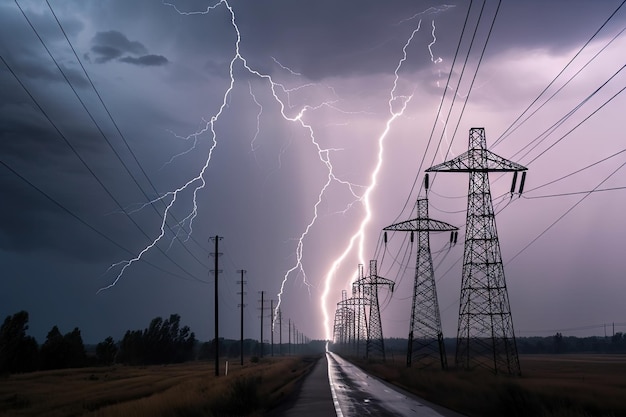The photo captures an intense lightning storm over a deserted two-lane country road. The sky is almost pitch black, attributed to the dense, dark clouds, with intermittent flashes from multiple powerful lightning bolts illuminating the scene. A particularly massive lightning strike is observed in the center of the road, splitting into a main bolt and several smaller forks.  On the left side of the road, a series of telephone poles with lines stretch into the distance. On the right, tall, reinforced metal power towers stand prominently, also extending as far as the eye can see. The image exudes a dramatic contrast between the dark, stormy sky and the bright, electric white of the lightning, highlighting the raw energy and power of the storm.